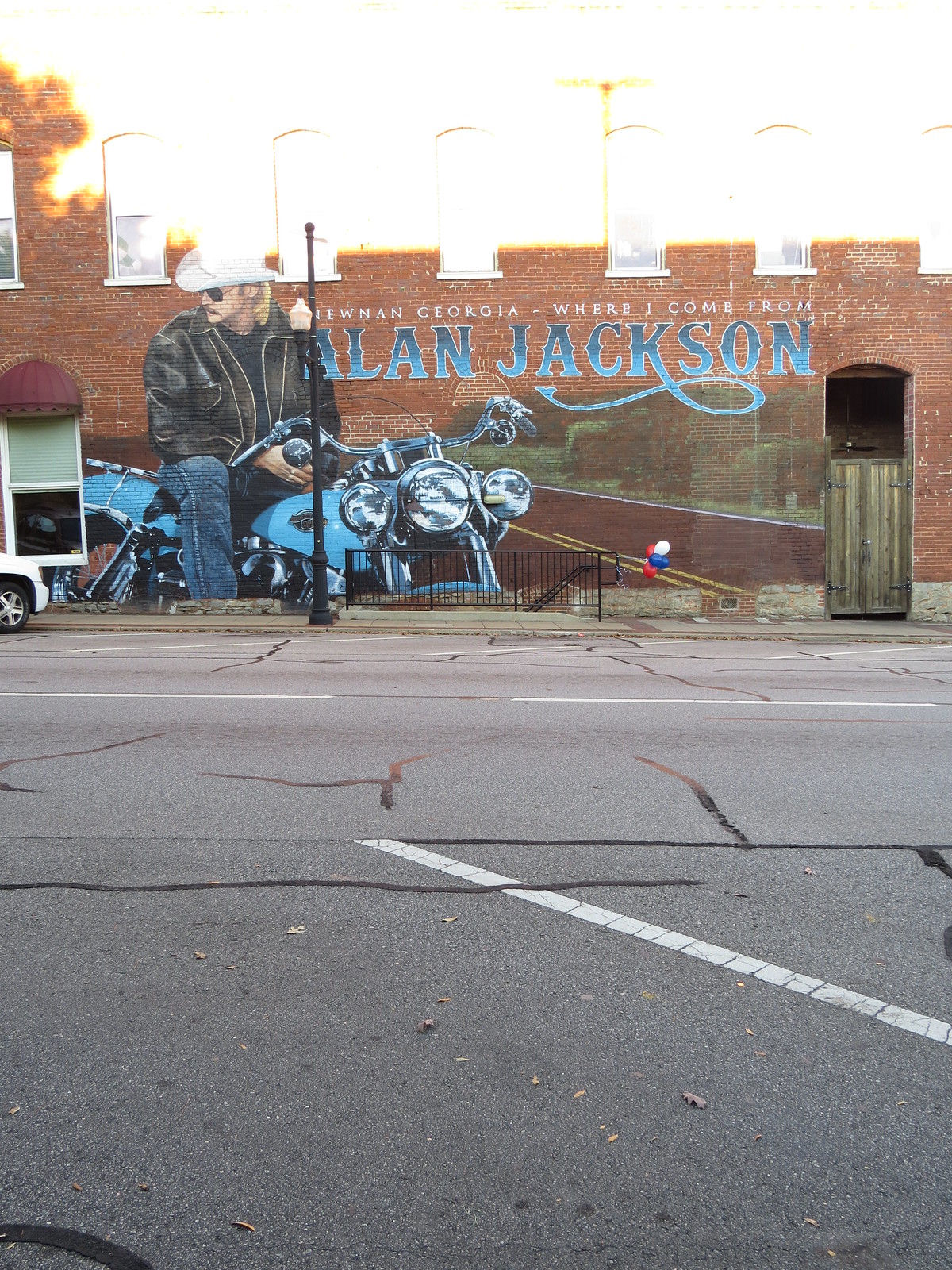This image captures a scene from a parking area on the side of a gray, cracked street in an urban setting, with the primary focus being a long, brownish-red brick building. The building, a couple of stories tall, features a prominent mural showcasing country music star Alan Jackson. The mural displays Alan Jackson wearing a leather jacket, white cowboy hat, jeans, and glasses, sitting on a blue motorcycle. His head is turned to the left side of the image. Beside the detailed portrait, the name "Alan Jackson" is written in a blue gradient, country-style lettering, with the distinctive 'K' looping back under the 'A.' The overall viewpoint is from the street, where white lines and black sealant for cover cracks are also visible, emphasizing the urban character of the scene. No cars are present in the image, drawing all attention to the vibrant mural on the building's side.